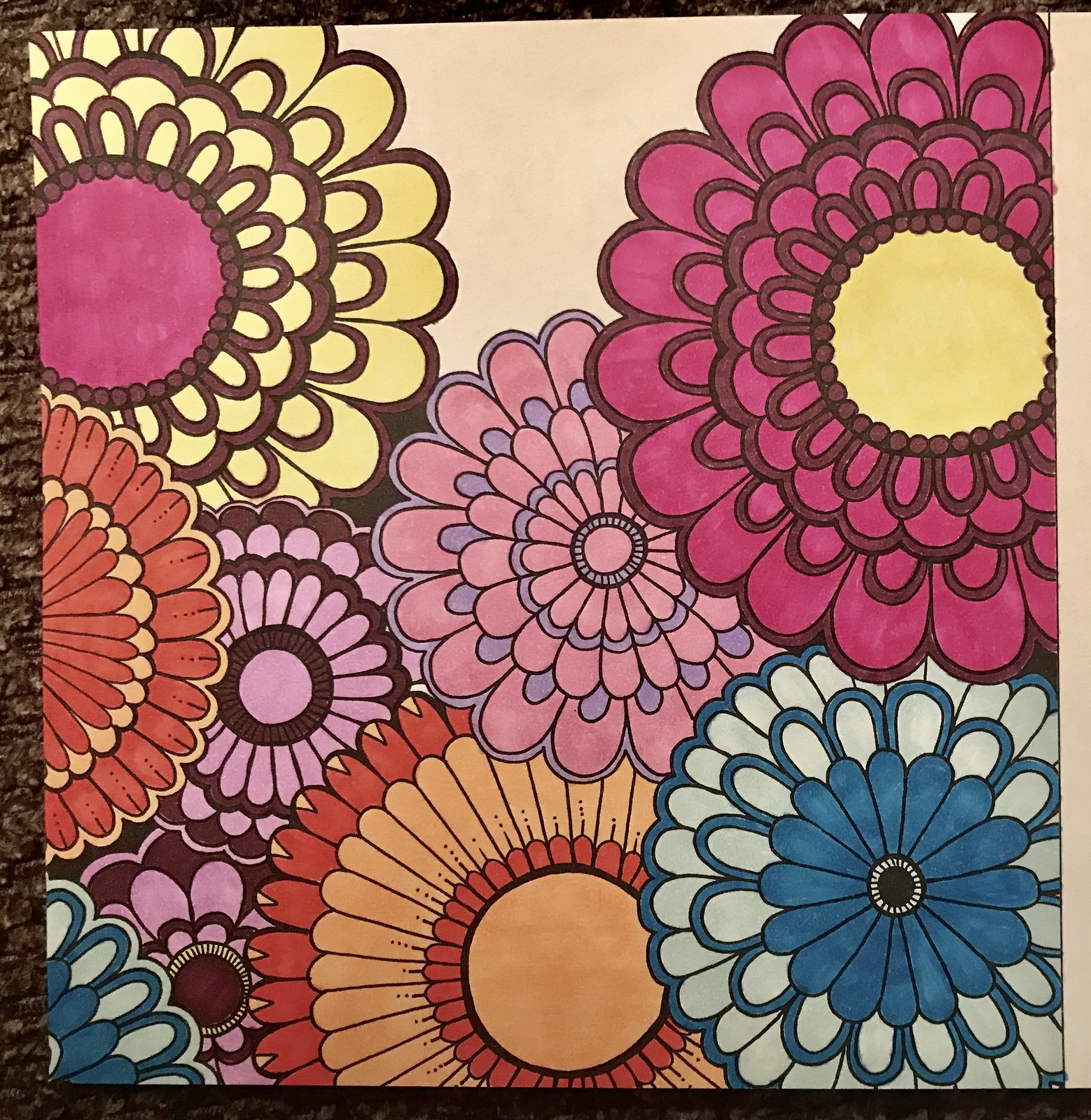An intricate, psychedelic artwork illustrates a vibrant array of sunflowers in a kaleidoscope of colors and patterns, evocative of the 1960s Beatles era. The composition features around nine or ten sunflowers, each uniquely varying in color and design. In the foreground, a sunflower with a bright yellow center and pink petals stands prominently, juxtaposed against a neighboring one with blue and white hues just below it. Scattered across the scene, other sunflowers showcase combinations of orange and dark orange, purple and pink, and various other captivating shades. Each flower is meticulously overlapping the others, creating a layered and dynamic visual effect. The intricate details extend to differing petal structures and vibrant color palettes, contributing to the overall psychedelic feel. The sunflowers occupy most of the space, but a section of the image reveals a cream-colored background, offering a subtle contrast to the vivid display of floral artistry.